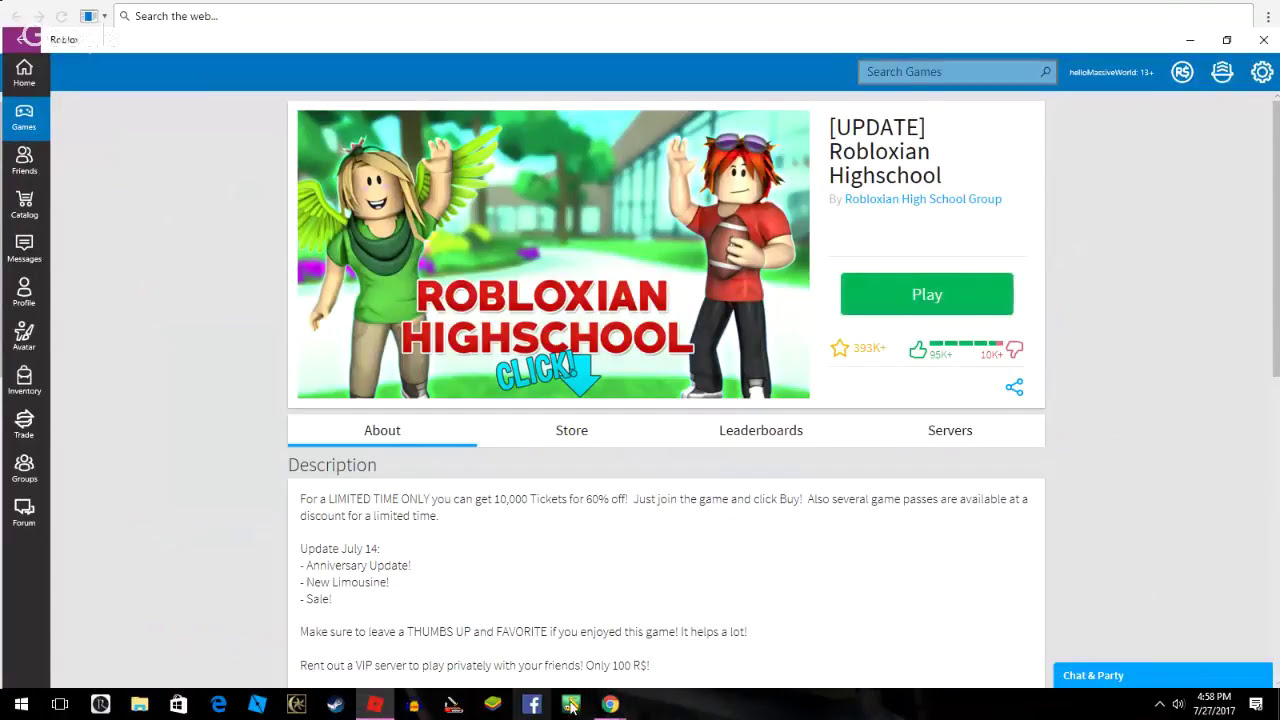The image is a detailed screenshot of a website interface for the video game "Robloxian High School." The screen is framed with a blue border at the top and a black one at the bottom. Centrally, the slide features two cartoon-like characters: a girl on the left with blonde hair, a green shirt, and angel wings, smiling and waving her hand, and a boy on the right with red hair, a red shirt, and sunglasses perched on his head, holding a football and also waving. 

In vivid red font between the characters, it says "Robloxian High School." Below this, a blue arrow points to text that reads "click below." The section underneath contains clickable tabs labeled "About," "Store," "Leaderboards," and "Servers." A description panel mentions updates like a "July 14th anniversary update" and a "new limousine sale," encouraging users to leave a thumbs up and favorite the game for support, and promoting VIP server rentals for private gameplay.

On the bottom right corner, there is a green play button, and just above it, in small text, it says "Update Robloxian High School."